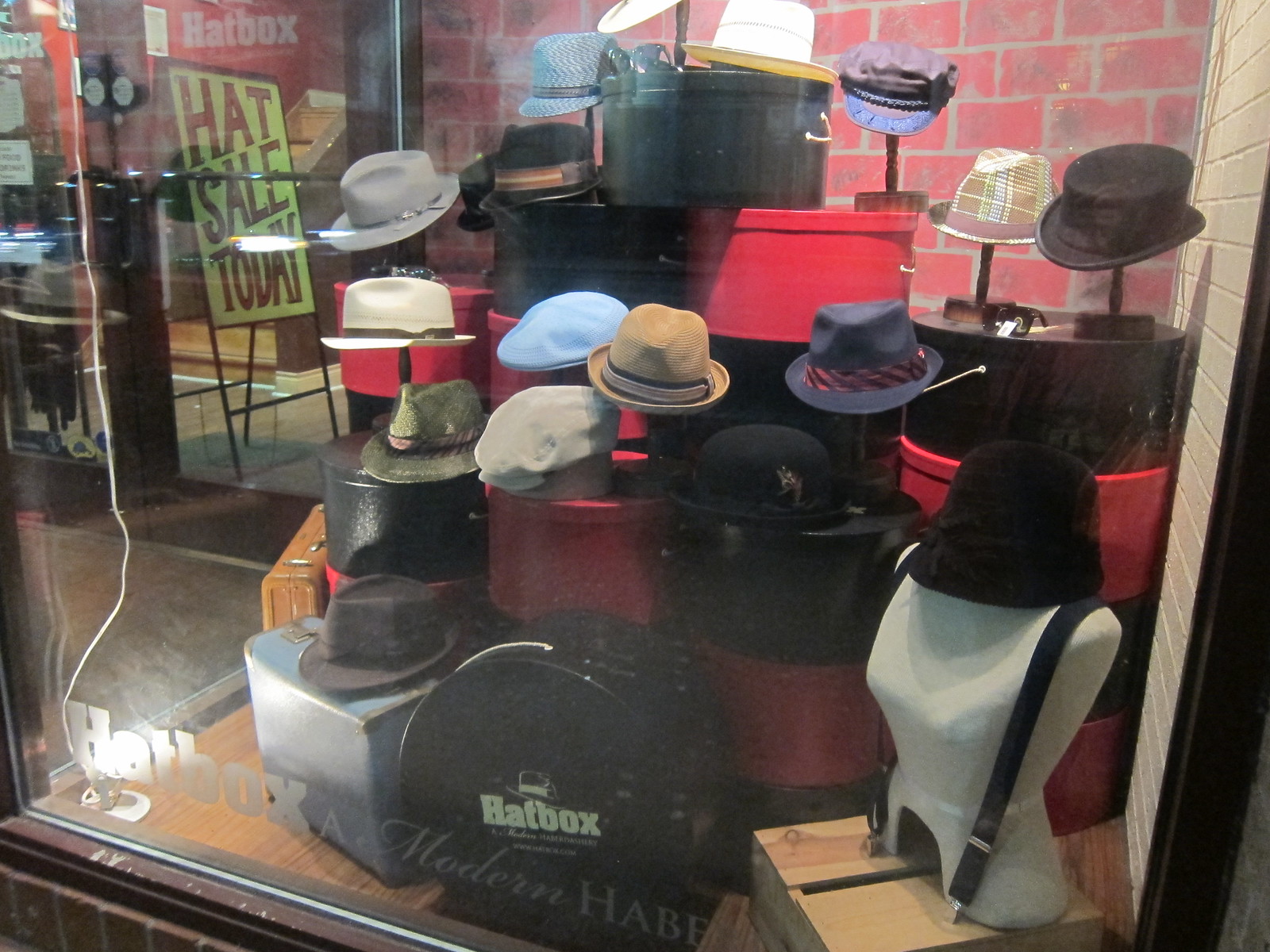This detailed photo captures the front of a modern haberdashery named "Hatbox," seen through a somewhat dirty store window adorned with red and brown trim that shows signs of wear, including white scratches. The lower portion of the store window features a brick wall and a large square glass pane with "Hatbox" written in silver paint at the bottom left corner. Inside the window display, an array of hats is showcased, ranging from top hats and Cuban-style hats to safari hats and mini top hats. The hats come in a variety of colors including black, brown, gray, white, light blue, and dark forest green. They are meticulously arranged on black and brown wooden stands, round and square display boxes colored in red and black, and atop suitcases—one brown and one baby blue. A white-gray mannequin also dons a hat, adding to the display's allure. In the background, a sign reading "Hat Sale Today" can be seen to the left. The entire display conveys a sense of nostalgia and elegance, fitting for a store specializing in fashionable headwear.